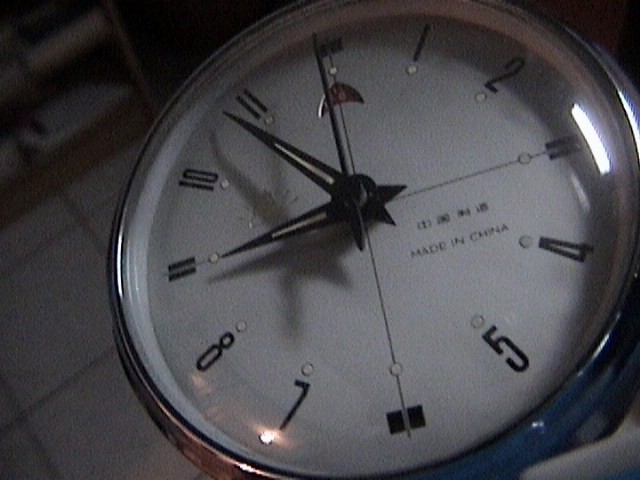The photograph is taken inside a dimly lit room, primarily capturing a close-up of a clock face that dominates around 70% of the image. The clock has a white background with bold black numbers in a long and narrow font. Hour and minute hands are black, while the second hand is metallic. Around the edge of the clock, a blue casing is partially visible. The clock face is marked with "Made in China" towards the bottom right, with additional, unreadable text possibly in Chinese above it. In the background, the bottom edge of wooden shelves stacked with paper is noticeable, and along the left edge of the image, the floor is visible with white square tiles, possibly marble, having horizontal and vertical lines that form a grid. The clock indicates the time is approximately 8:54.